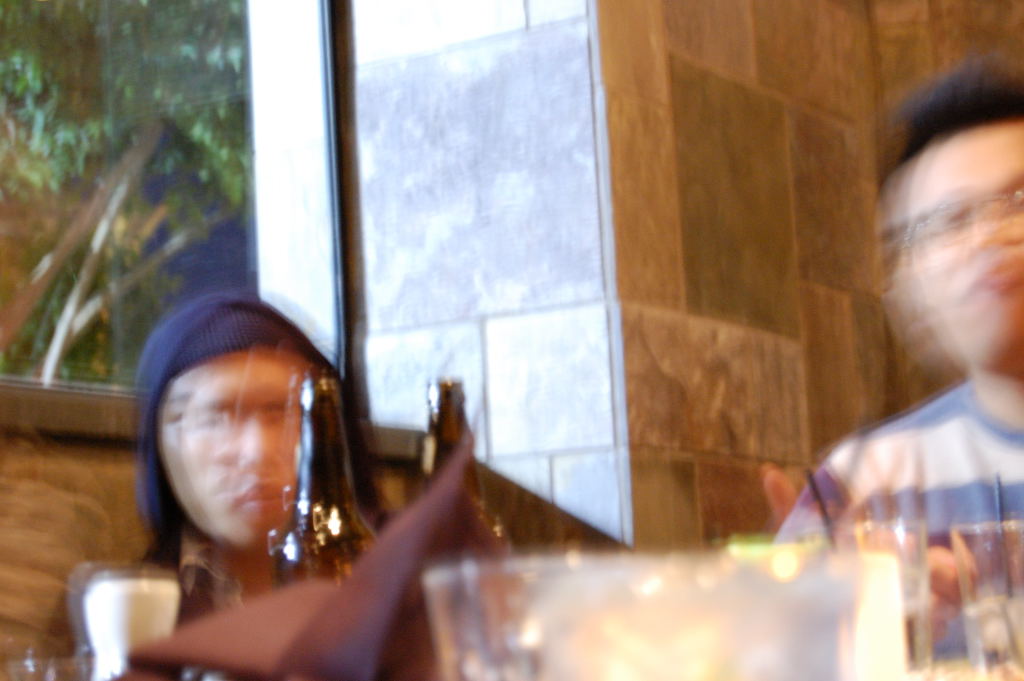The image is an indoor color photograph taken from a very low angle, almost level with the surface of what appears to be a dining table. Although the table itself is not visible, it is covered with various drinking glasses and brown beer bottles. An illuminated candle in the foreground, close to the center of the frame, casts a warm glow. The photograph captures a horizontal view across the table at two people sitting in the background.

The two individuals are blurry, indicating some motion when the photograph was taken, resulting in a ghosting effect with lighter repeats of their faces. The person on the right, pouting with short black hair and glasses, is wearing a light blue and white striped t-shirt. The individual on the left has a neutral expression and is dressed in a black hoodie and a black cap, resembling a toque, with a collared t-shirt peeking out from underneath.

Behind the person on the left, a large window is visible, showing a couple of branches and some green foliage outside, suggesting a restaurant setting. The exact time of day is ambiguous due to the lighting, which appears both bright and dim at the same time. The background also features tiled walls of light brown, green, and grey shades. There is no visible text in the image, only the subtle hints of an intimate dining environment.